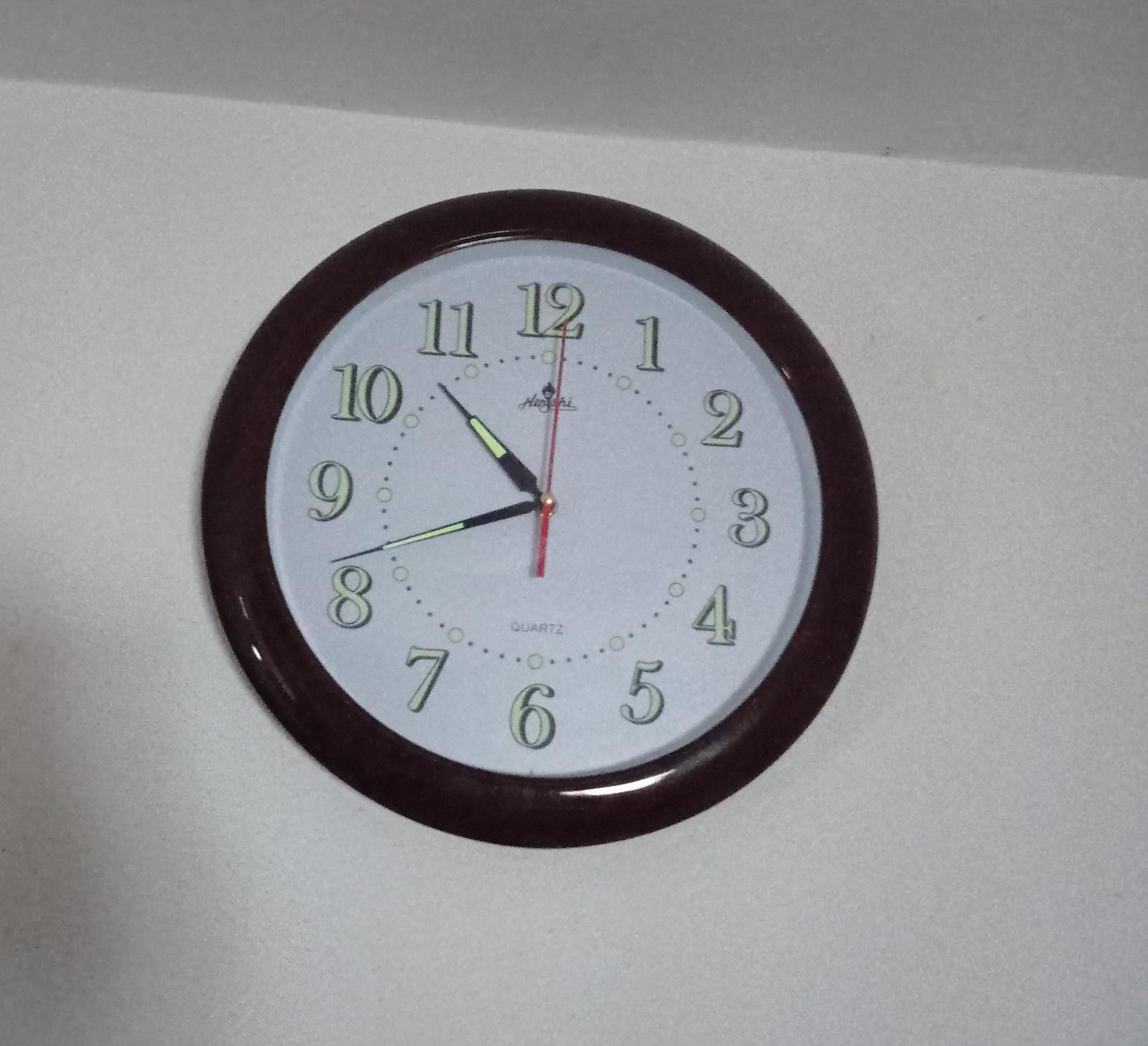This image captures the upper portion of a wall where it meets the ceiling, with a partial view of the ceiling itself. Prominently featured on the wall is a large, dark clock, possibly black or brown in color. The clock's face has a white inner section where the numbers are displayed. These numbers are styled in bubble letters with a light yellow or possibly cream hue, and they are slightly shaded for a subtle 3D effect. Encircling the numbers is a decorative ring composed of numerous dots. The clock face also includes the text "Quartz" and a brand name, which is somewhat difficult to read but appears to be "850."